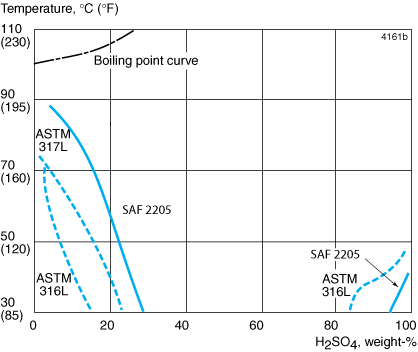The image is a detailed chart set against a white background, featuring a graph that highlights temperature data in both Celsius and Fahrenheit. The y-axis on the left indicates temperature values starting from 30°C (85°F) up to 110°C (230°F), with labels at each interval: 30 (85), 50 (120), 70 (160), 90 (195), and 110 (230). The x-axis across the bottom is labeled as H2SO4 weight percentage, ranging from 0 to 100. The graph is segmented by a grid composed of intersecting lines forming squares. A blue dotted line spans the graph horizontally, with a bold black line marked as the "boiling point curve," specifically for SAF 2205. The overall graphic presents a clear visualization of the boiling point in relation to varying H2SO4 concentrations, emphasized by the use of blue and black lines for different data sets.